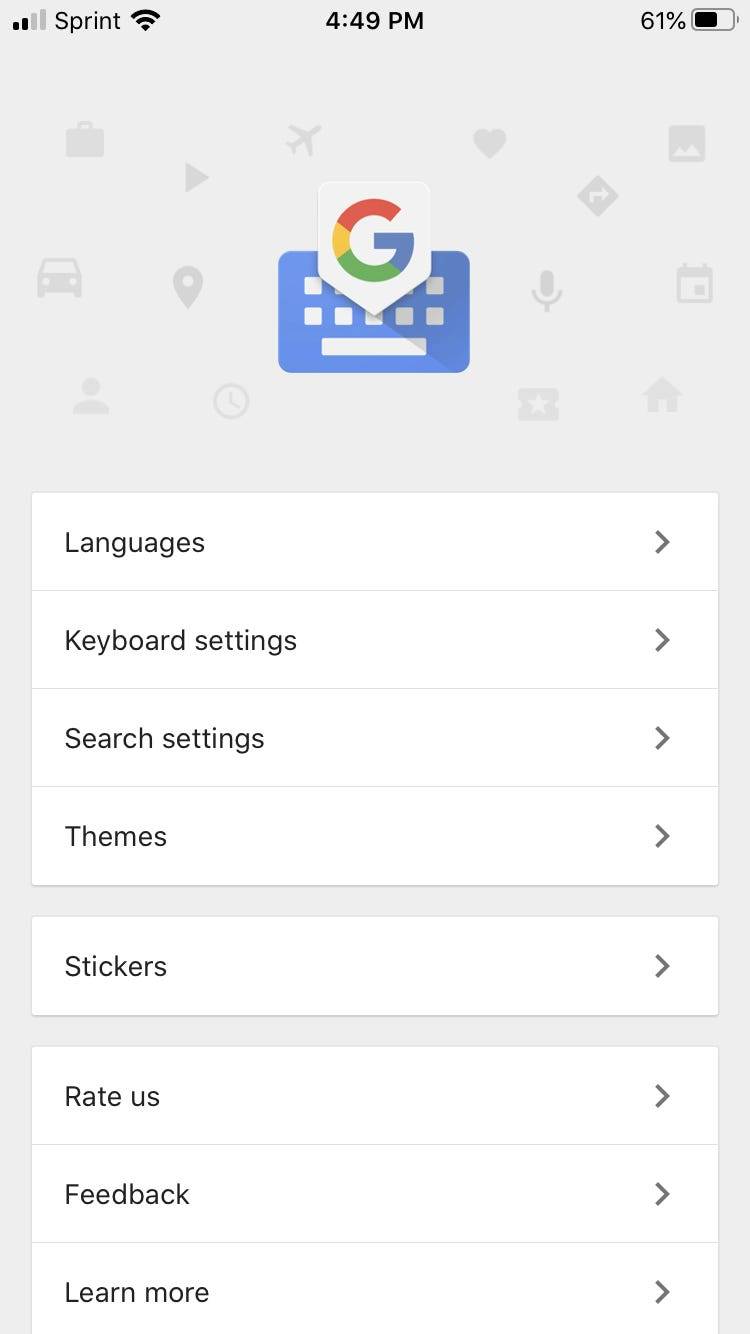This is a detailed screenshot captured from a mobile device. Starting at the top left corner, there is a data signal indicator showing two out of four bars filled, denoting moderate signal strength, with the Sprint logo next to it. In the center, a Wi-Fi symbol is displayed, and the time reads 4:49 PM. On the top right corner, the battery status shows 61% with an accompanying battery icon.

The screenshot displays a Google page, most likely Google Translate, identifiable by the colorful "G" of the Google logo over a blue graphic of a keyboard. Surrounding the logo are various gray icons depicting different objects and actions, such as a car, play button, airplane, heart, microphone, house, and calendar, adding a decorative touch.

Beneath the logo, there is a series of navigation options listed from top to bottom as follows: Languages, Keyboard settings, Search settings, Themes, Stickers, Rate us, Feedback, and Learn more. Each of these options is accompanied by a right-pointing arrow (>) indicating that they can be expanded for more information.

The overall color scheme of the page is minimalistic, primarily featuring white buttons and sections against a light gray background, giving it a clean and neutral aesthetic.